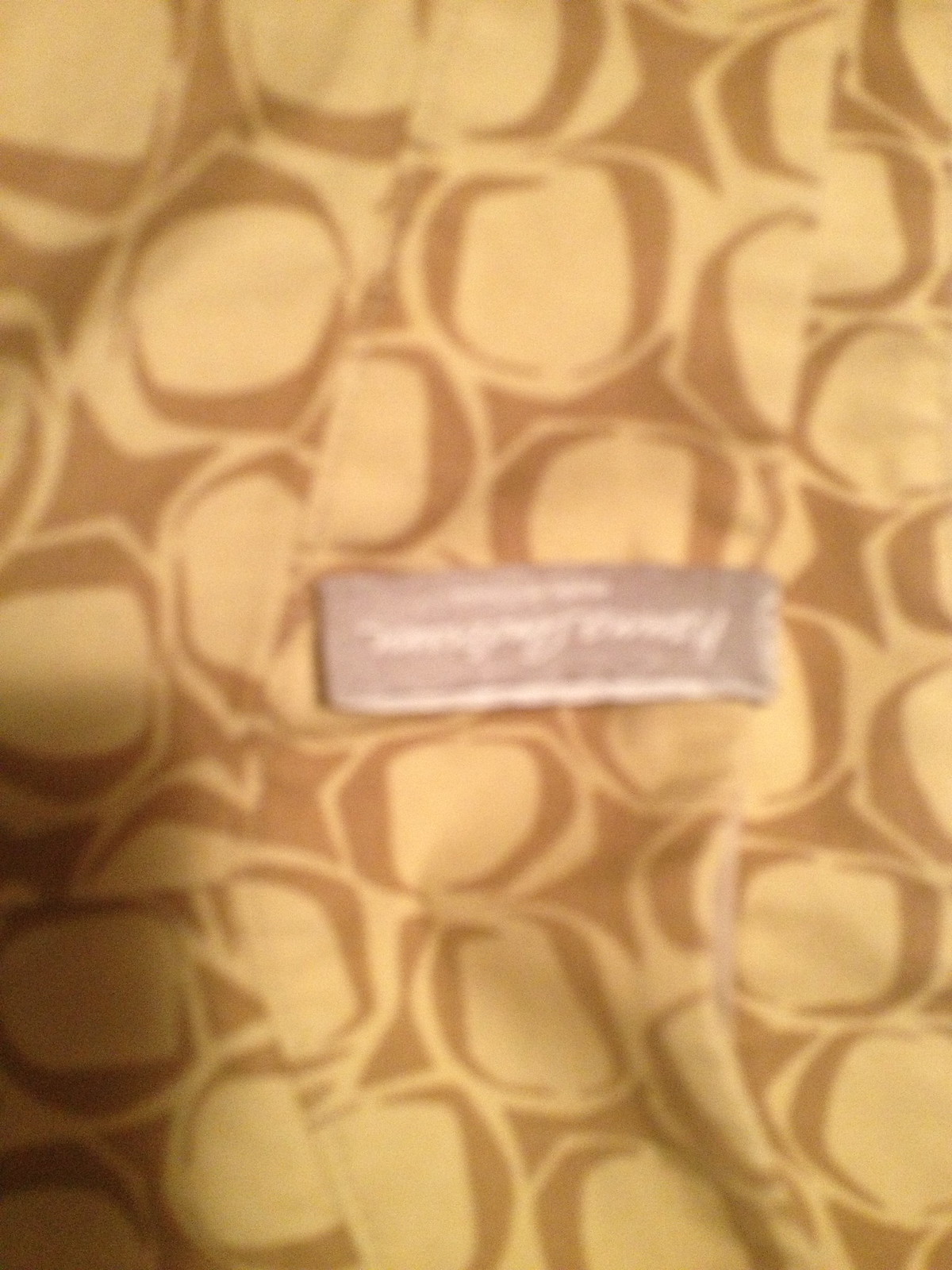This is a highly blurred image with an overall low resolution, making it challenging to decipher details. At the center of the picture, there is a rectangular, silver-colored label, possibly a tag. The label appears to be upside down and it is difficult to read the text, though it may say "Brooks Brothers" in white or pearl-colored letters with some light reflecting off it. The fabric background of the label is either a piece of clothing or a cloth item, displaying a yellow or off-white color with an intricate, brown pattern resembling interlocking 'C's or emblem-like designs. The general background of the image features a blend of yellow and brown hues with some artistic designs, contributing to the overall fuzzy and indistinct appearance.